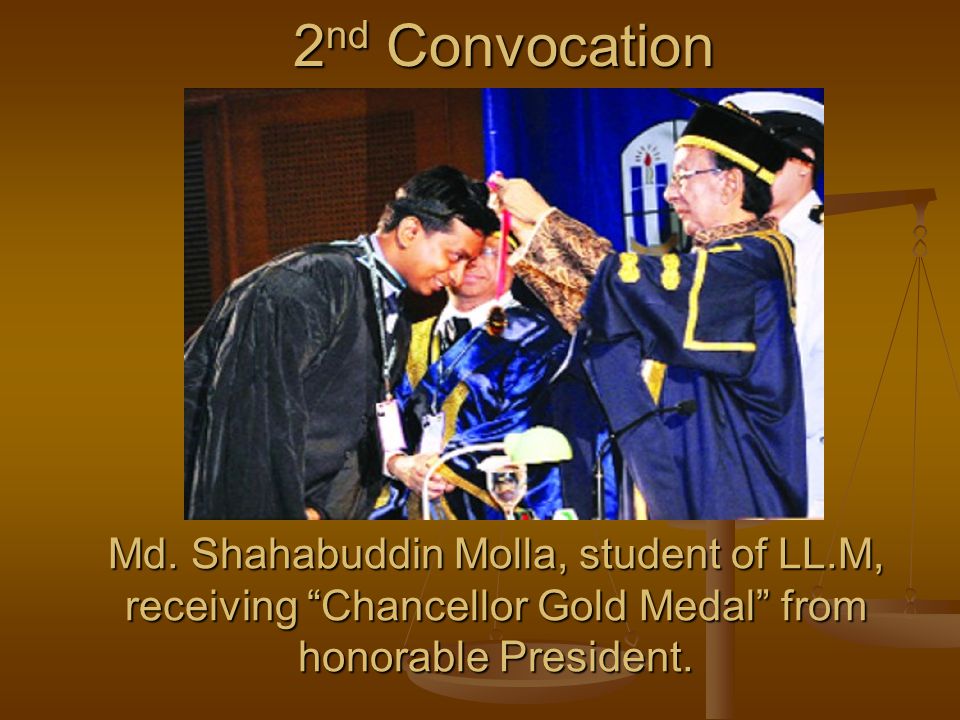The image is a PowerPoint slide with a background featuring gold brass-colored scales of justice. Topped with the title "Second Convocation" in gold or light beige lettering, the slide centers on a photograph depicting a graduation ceremony. In the photo, a graduate in a black gown is bent slightly forward, receiving a Chancellor's Gold Medal from a distinguished figure in a blue robe adorned with gold bars and accessories, presumably the honorable president. The professor wears a black graduation cap while placing the medal around the neck of M.D. Shahabuddin Molla, identified by the text below as a student of LLM.